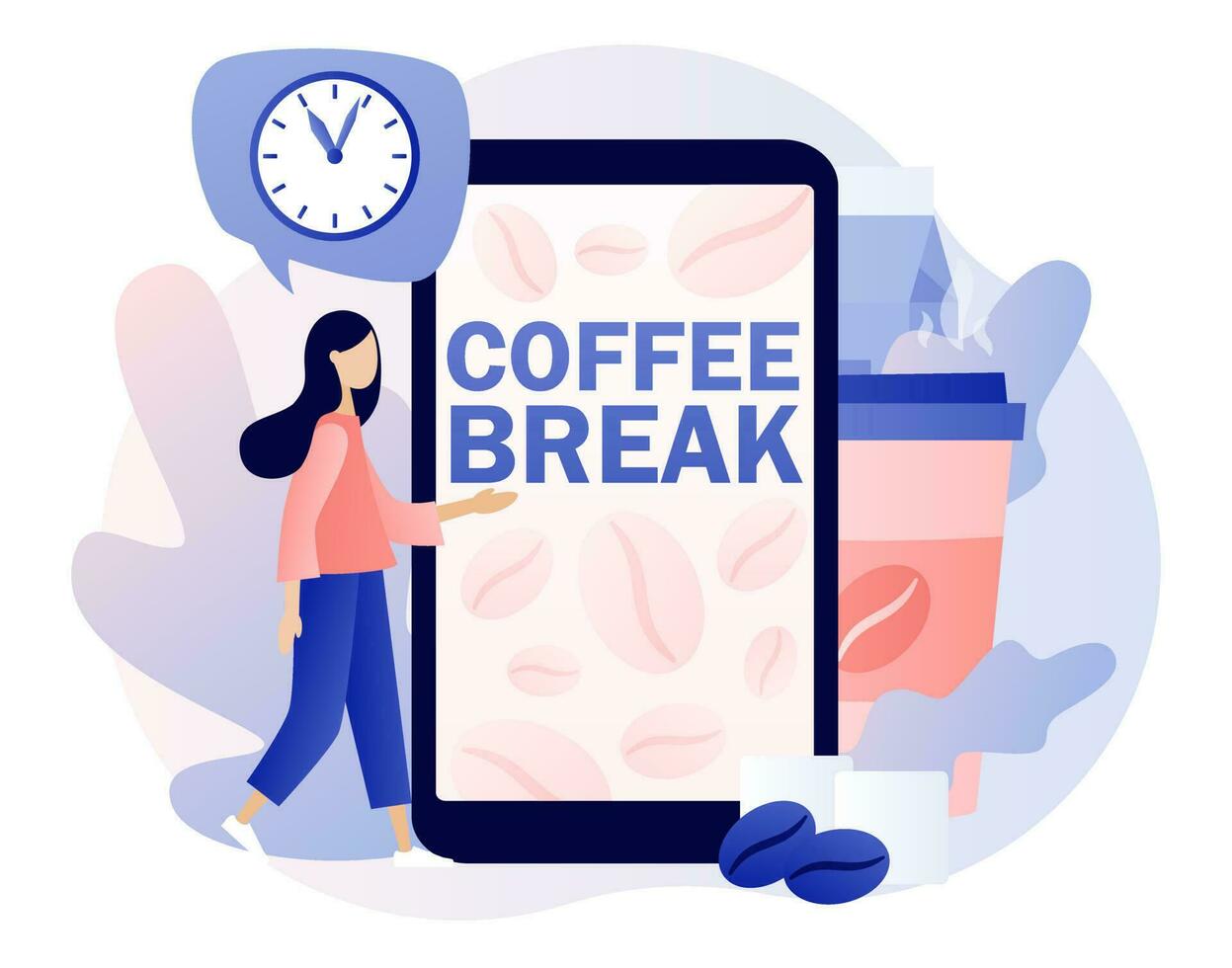The image is a digital illustration set against a light lavender background. Central to the image is a cartoon woman with black hair, dressed in blue pants, a pink long-sleeve shirt, and white shoes. She stands to the left side of a large depiction of a cell phone. Above her head, a blue speech bubble contains a clock showing nearly 1:00, emphasizing a sense of urgency or break time. The text "coffee break" is prominently displayed in an indigo or purplish font on the phone screen. To the right of the woman and the phone is a large cup of coffee with a blue lid, featuring a logo of a diagonal circle with a white line passing through it. Below the phone are two large blue coffee beans, suggesting time for relaxation and refreshment. Overall, the image uses a mix of pink, blue, white, black, and gray colors to create a cohesive and inviting scene.